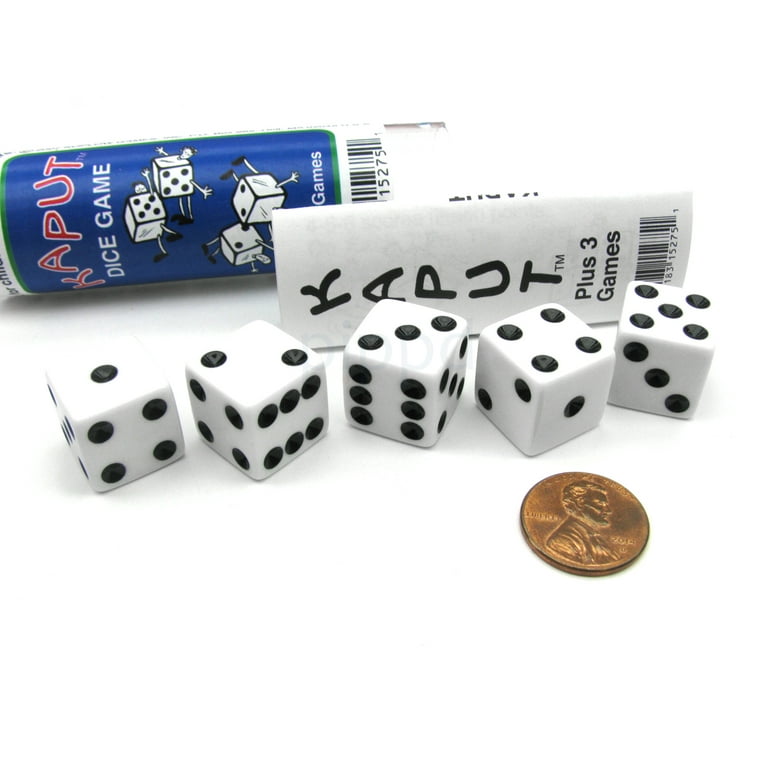This photograph showcases the contents of a dice game against a plain white background, resembling a product image one would find on a retail site. Central to the composition are five white dice with black dots, arranged in a row from left to right. The faces of the dice display the numbers in ascending order: 1, 2, 3, 4, and 5. A penny, placed heads up, lies just in front of the fourth and fifth dice, serving as a size reference. Behind the neatly ordered dice rests a folded instruction booklet bearing the title "Caput Plus 3 Games" and a visible barcode. Further back, the tubular container designed to hold the dice and instructions stands upright, featuring the label "Caput Dice Game" along with playful cartoon images of dice with arms and legs.